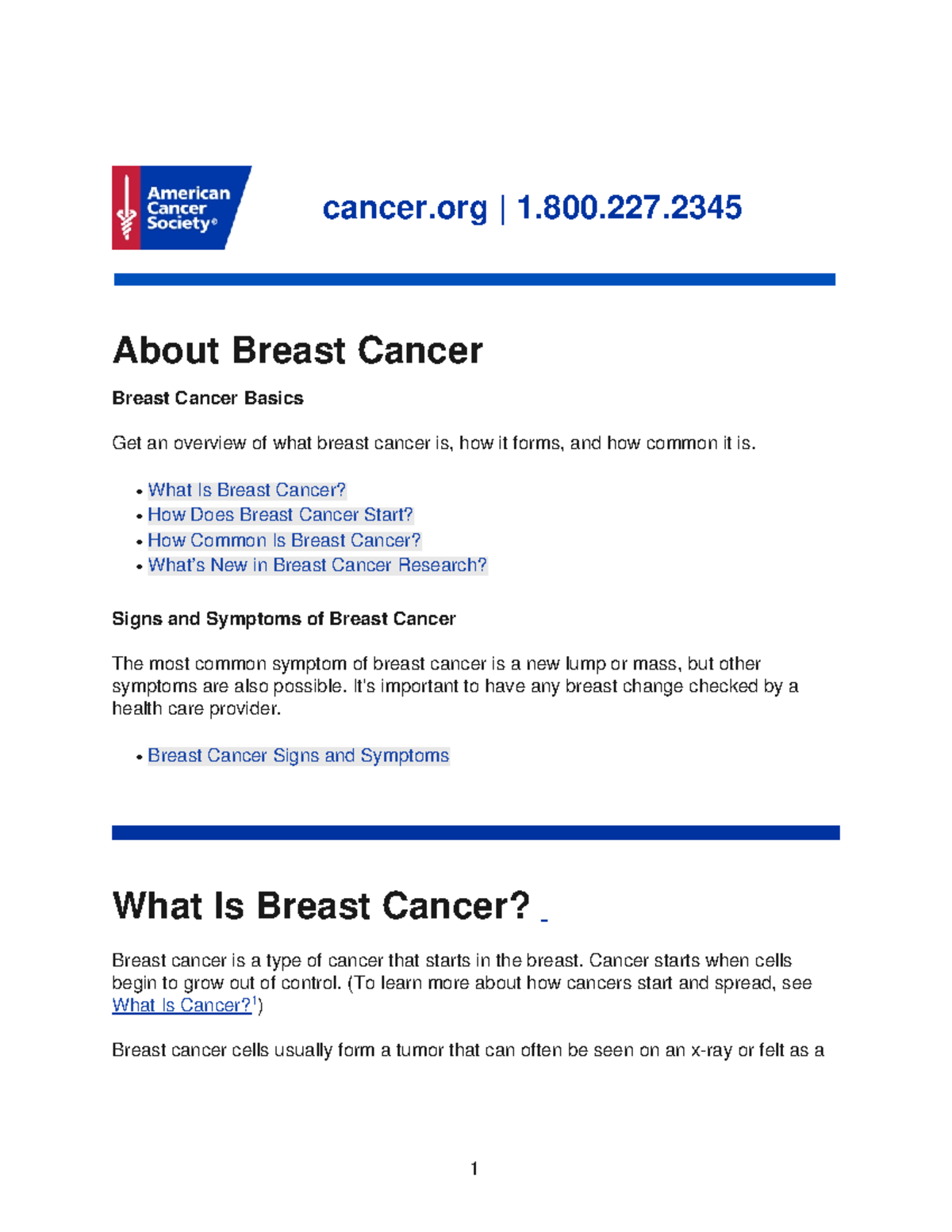This is a detailed screenshot from the American Cancer Society's website. In the top left corner, the American Cancer Society logo is prominently displayed, adjacent to the URL "cancer.org" in bold blue text. Beside the URL, the contact number "1-800-227-2345" is also presented in bold blue text. Below these elements, a horizontal blue line spans the width of the image, providing separation from the main content.

Underneath the blue line, the heading "About Breast Cancer" appears in black text. Directly below, a subheading "Breast Cancer Basics" is followed by a brief description in smaller black text, stating: "Get an overview of what breast cancer is, how it forms, and how common it is."

The section also offers four clickable options in blue text links: "What is breast cancer?", "How does breast cancer start?", "How common is breast cancer?", and "What's new in breast cancer research?".

Further down, another heading "Signs and Symptoms of Breast Cancer" is displayed in black text, followed by a short paragraph describing these signs and symptoms. A blue text link reiterates "Breast Cancer Signs and Symptoms" for further reading.

Another horizontal blue line separates this section from the next. Below it, a larger black heading declares "What is Breast Cancer?" followed by a brief introductory paragraph. Within this paragraph, a blue clickable link labeled "What is Cancer?" offers additional information. The image ends with the start of another paragraph that is mostly cut off and not fully visible.